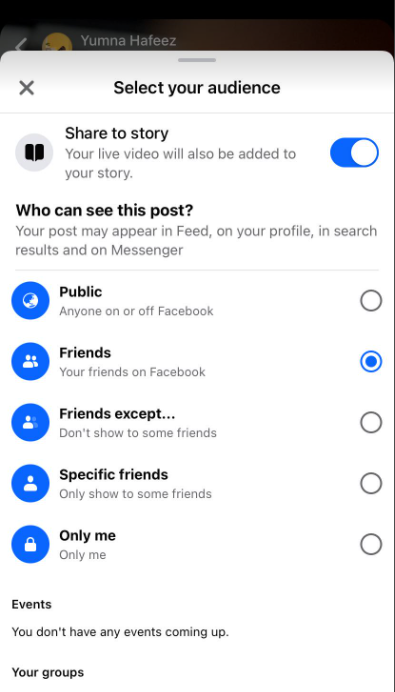The image depicts a Facebook mobile interface for selecting the audience of a live video or story. The screen has a white background with black or gray font. In the upper left corner, there's an 'X' icon to exit the menu. The header reads "Select Your Audience,” and below it, there’s a section indicating that your live video will also be added to your story, which is toggled on.

The section titled "Who can see this post?" explains that your post may appear in the feed, on your profile, in search results, and on Messenger. The visibility options include:

1. **Public**: Anyone on or off Facebook.
2. **Friends**: Your friends on Facebook (currently selected, indicated by a blue circle on its right side).
3. **Friends except...**: Allows you to exclude certain friends.
4. **Specific friends**: Limits visibility to a select group of friends.
5. **Only me**: Makes the post visible only to you.

Further down, under "Events," it says you don’t have any upcoming events. The "Groups" section follows but is not populated with any specific information in the image.

At the bottom, it shows the profile name "Yumna Hafeez," implying that this is the person setting the audience for their live video or story. A gray overlay indicates that this menu is currently active.